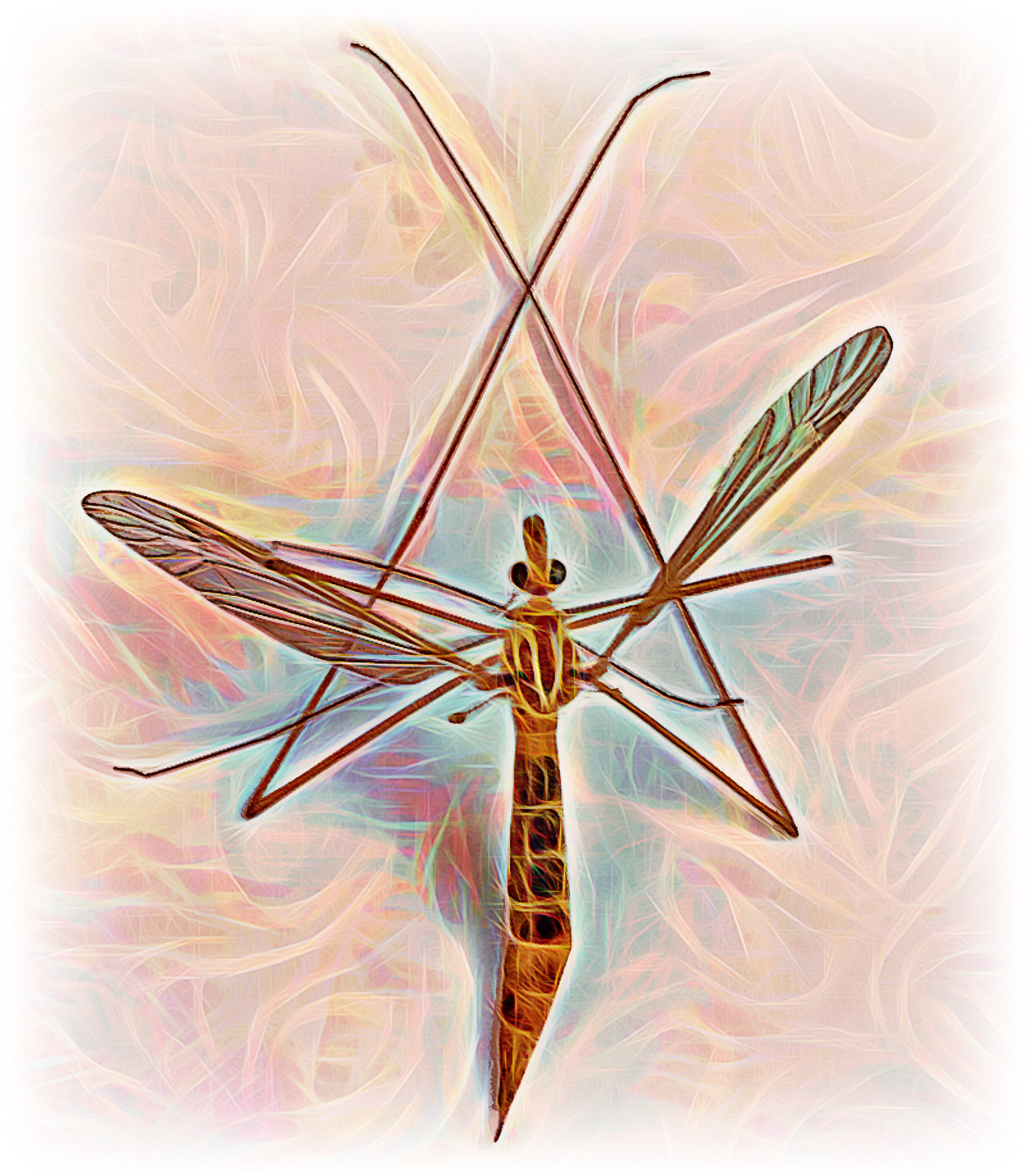The image is a rectangular painting, approximately six inches high and four to five inches wide, bordered by a soft, fade effect that gives it a cloud-like appearance. The central figure is an insect resembling a dragonfly, with a highly geometric and somewhat awkward appearance. The insect has an elongated, orange body, brown tail, and large, bulbous black eyes that protrude on either side of its head. Its legs are notably long and angular, crossing in front and making shapes reminiscent of a star or a teepee, while other legs extend outwards and then bend back in.

The dragonfly’s wings, one of which appears slightly broken, are pink and green with translucent inner sections supported by veins. They cross behind the insect, forming an X shape. The entire scene is bathed in a glowing light teal color, enhancing the insect's otherworldly glow. The background features a dynamic swirl of pink, blue, green, and orange hues, creating a vibrant and surreal setting that accentuates the insect’s unique and striking presence. The painting's overall effect is one of both vivid detail and ethereal beauty, capturing the viewer’s attention with its intricate and colorful design.